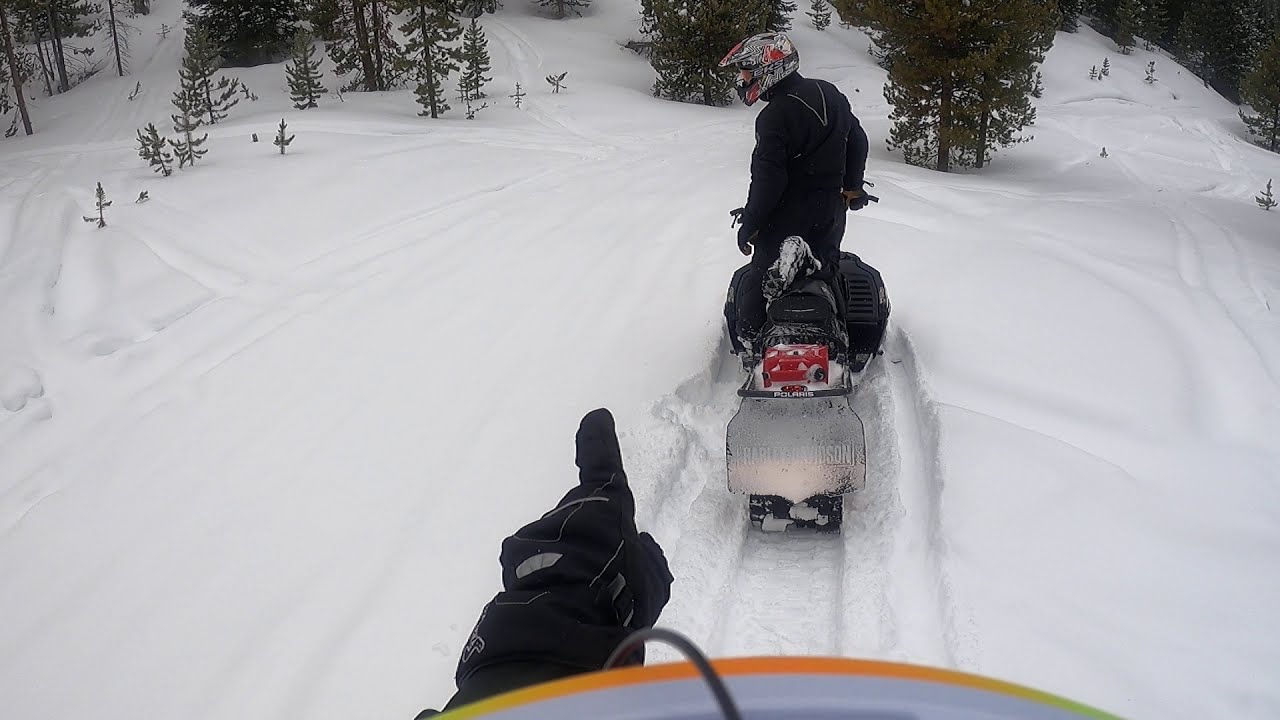In this vivid outdoor scene set on a snow-covered hill, a man is prominently riding a silver Polaris snowmobile with a black storage box at the back. Dressed in a black jacket and black pants, he dons a colorful helmet embellished with red and white patterns. He is heading down the hillside, surrounded by a pristine blanket of white snow. His gloved hand extends forward, pointing towards the foot of the hill. In the foreground, lush green pine trees stand tall, and the setting hints at a snow sports resort. Behind the man, the circular front part of another vehicle peeks out from the top of the hill. The image, captured from a first-person perspective, suggests an overcast day, brightened by the expansive snowy landscape. The scene is alive with the thrill of winter adventure and is marked by the iconic "Polaris" branding on the snowmobile, emphasizing the exhilarating activity unfolding in this picturesque winter wonderland.